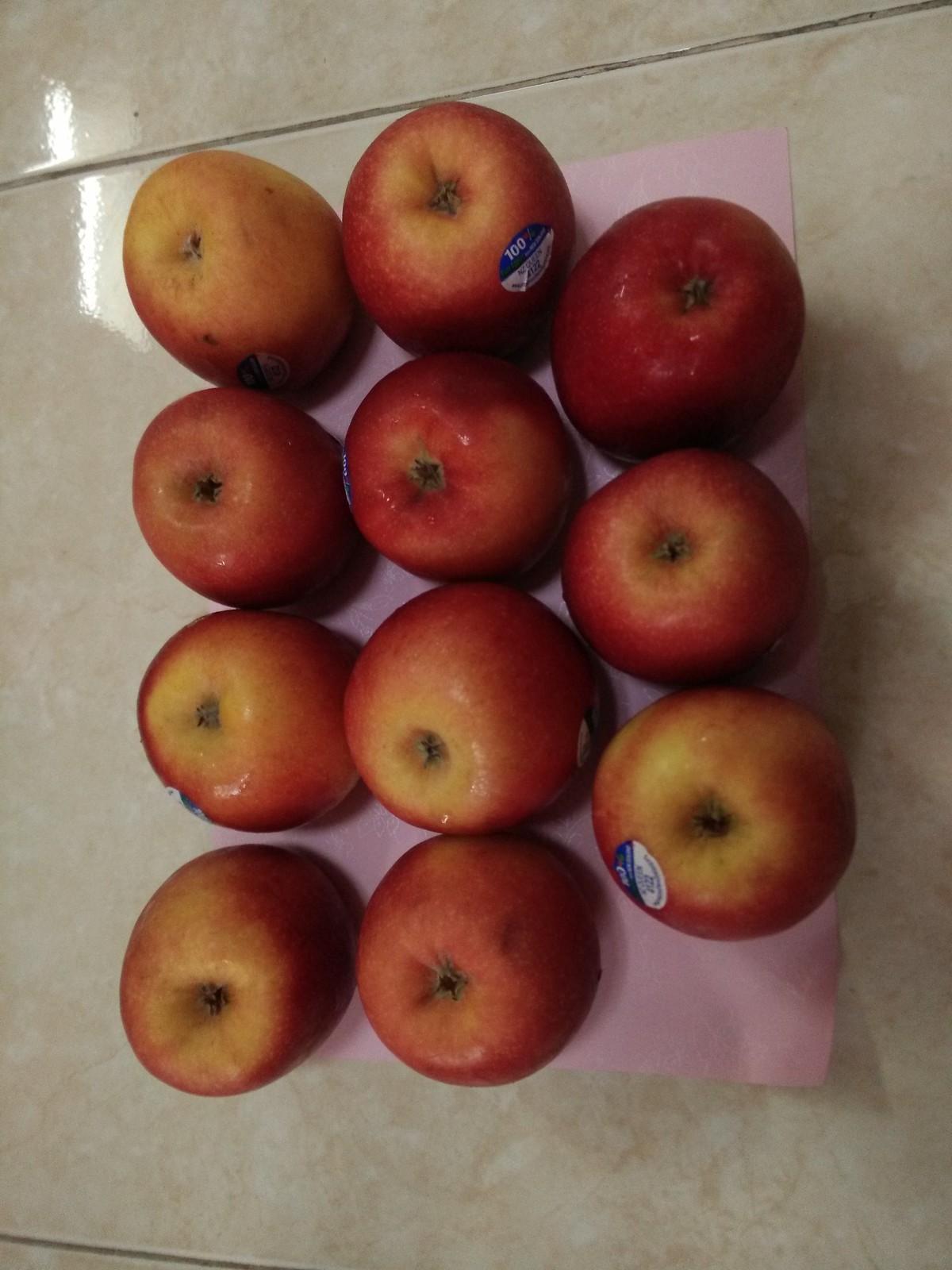The photograph showcases a neatly arranged collection of eleven recently washed apples, seen from a top-down perspective. The apples are organized into three vertical lines; the first and the middle lines each contain four apples, while the third line contains three. These apples, likely Gala apples, are predominantly red with varying patches of yellow, particularly on the base. The image captures the apples resting blossom side up on a pink paper towel, which is laid out vertically. The apples glisten slightly, indicating they are still damp from washing. Some have small, horizontally split oval stickers in navy blue and white, denoting type or origin, although the specific details on the stickers remain indistinct. Below the towel, the apples sit on a beige ceramic tile surface adorned with faintly darker striations. A grout line, in a dark grey-brown hue, runs diagonally from left to right towards the top and bottom edges of the image, adding a subtle, textured detail to the background.